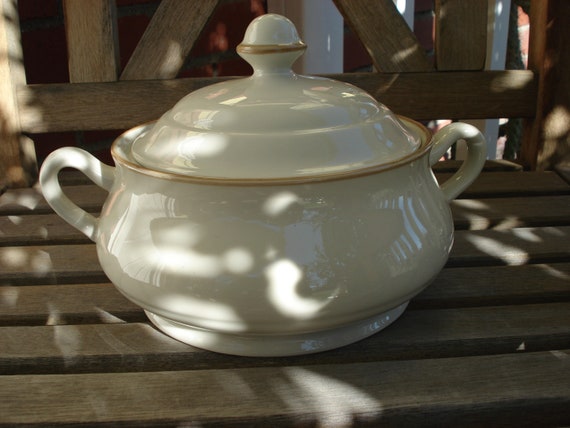This image showcases a fine china terrine, exquisitely designed for elegant occasions such as Thanksgiving or Christmas celebrations. The terrine is a roundish, off-white piece with a refined porcelain finish. It features two sturdy handles on either side that resemble, but are thicker than, teacup handles. The rim of the base is adorned with a delicate goldish-brown border, matched by similar accents on the dome-shaped lid. The lid includes a pronounced ridge midway up, culminating in a knob topped with a goldish-brown tip, designed for easy lifting. The terrine sits on a wooden bench with wide, dark wood slats running horizontally, to which the seat back is partially visible. The contrast of the terrine’s soft colors against the dark wood emphasizes its elegant design and craftsmanship.